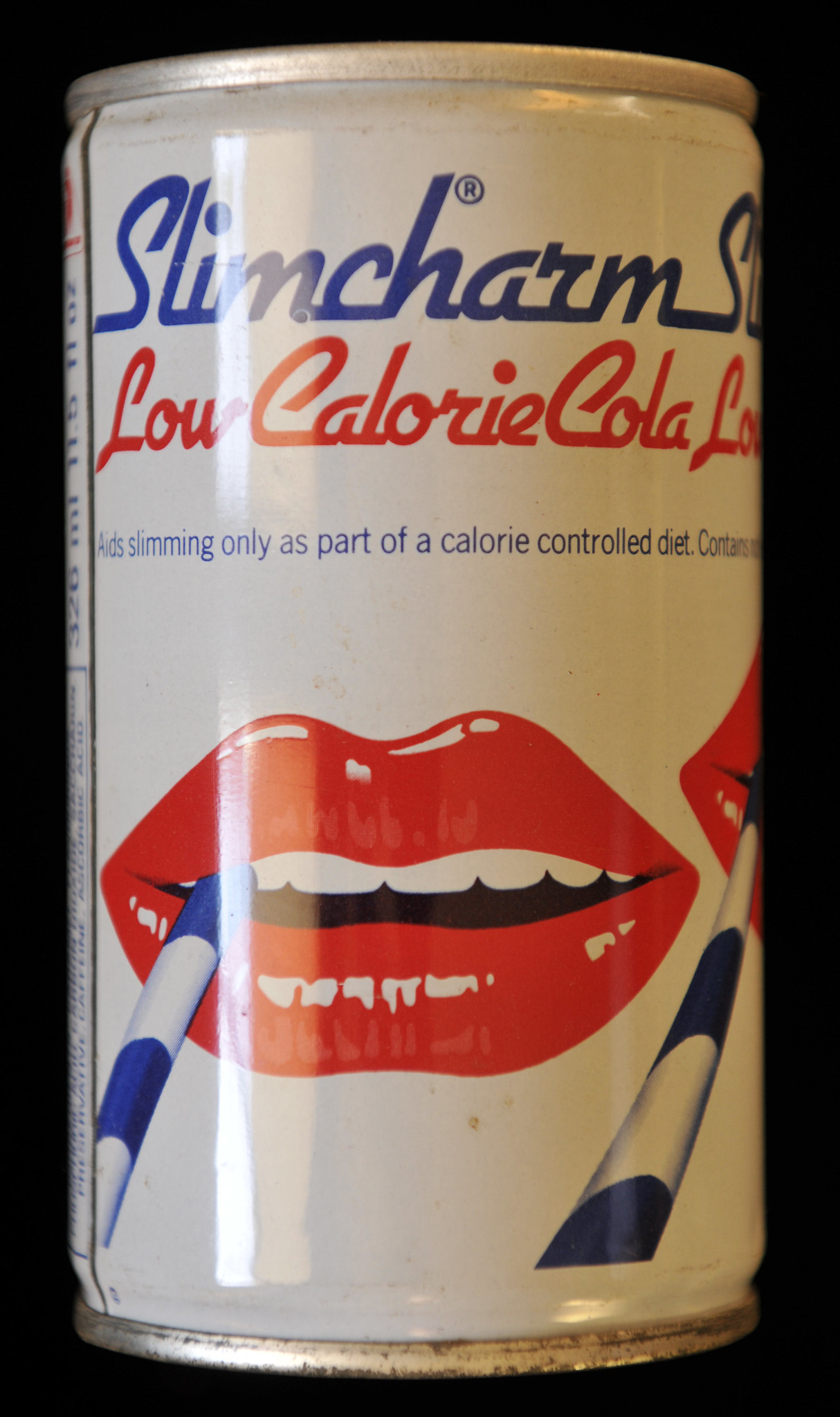The image showcases an aluminum can designed as a beverage container. The can, predominantly white, features a top-title that reads "Slim Charm" in a vivid combination of blue and red lettering. Just below this, the descriptor "Low Calorie Cola" is prominently displayed. Further down in a blue font, the text declares, "Aids Slimming Only as Part of a Calorie Controlled Diet." Adding a touch of visual flair, there is an illustration of slightly open red lips revealing white teeth, with a striped blue and white straw positioned to the side of the lips. The entire can is set against a stark black background, which enhances the contrast and highlights the can's details.